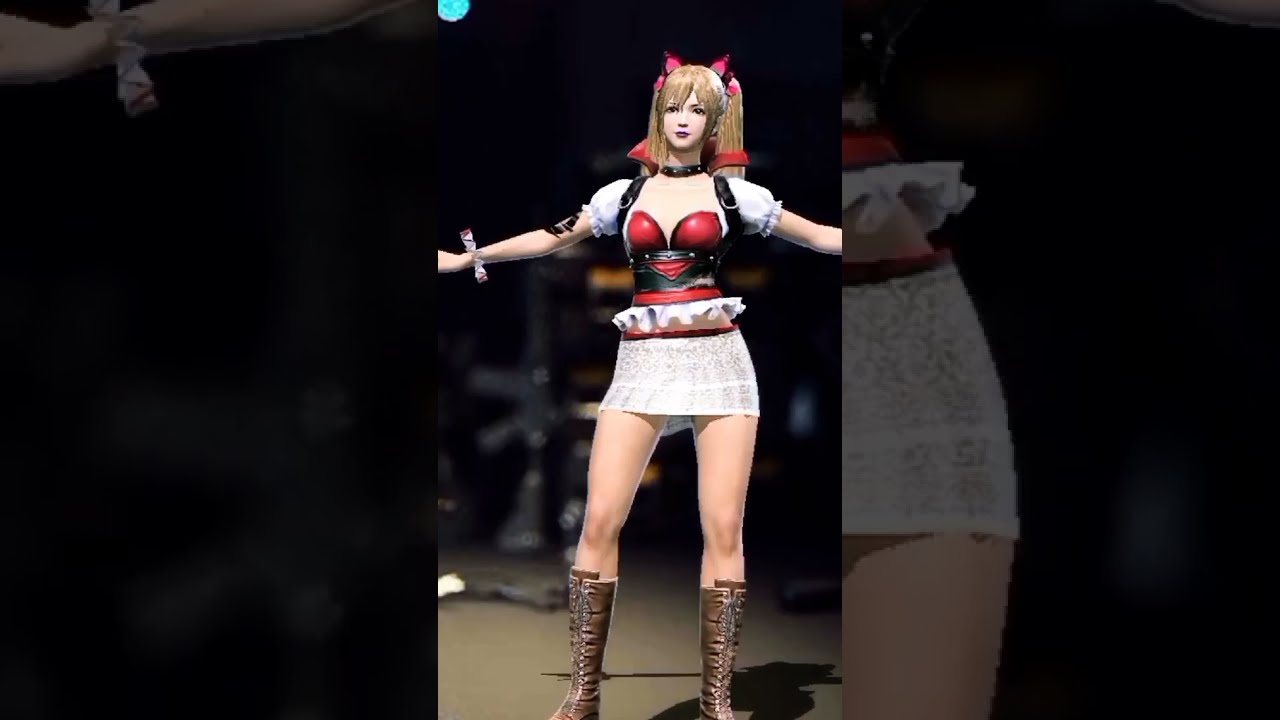The image in question appears to be a screen capture from a video game or animation, presenting a central female character depicted in a cartoonish or slightly anime style. The character stands in the middle of the frame with her arms outstretched to her sides, creating a balanced and open stance. She has light skin, and her light brown or dark blonde hair is styled into pigtails with pink bows, topped with pink cat ears.

Her attire is detailed: she wears a lacy short white skirt resembling a tutu with a little more decoration around the edges, paired with tall brown boots that lace up to just below her knees. She dons a striking red leather corset featuring a black strap around the waist and silver buckled straps on her shoulders. Underneath the corset, she sports a short-sleeved white top with frilly edges that almost reach her elbows.

The background of the image is somewhat blurred, possibly showing a carpeted floor, and it gives the impression of being an indoor setting. The main image is repeated behind the character in larger, darker, and more zoomed-in sections focused around her midsection. The color palette includes shades of tan, brown, white, red, black, and light blue. Notably, the character has rosy cheeks and red lips, emphasizing a lively and vivid aesthetic without any accompanying text.